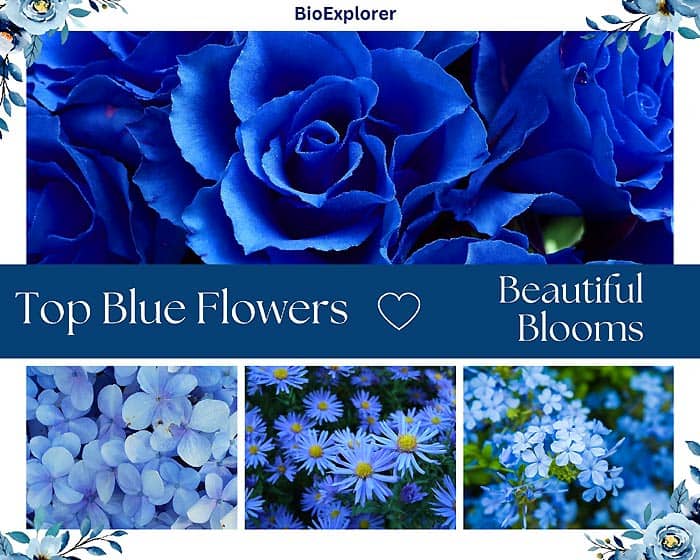The image is a rectangular digital collage designed as a banner or slide for a blog. The top and bottom sides of the image are twice the length of the left and right sides. The collage is bordered by a solid white frame, with each corner—top left, top right, bottom right, and bottom left—featuring a hand-drawn blue flower of a different species. The center of the image is spanned by a dark blue banner with white text reading, "Top Blue Flowers, Beautiful Blooms," and includes a small white heart icon. The largest photograph, occupying the entire top half of the collage, is a close-up of a blue rose set against a black background. Below this, the bottom half of the collage displays three different photographs of various blue flowers, each within its own square frame. Near the top of the image, in the white space, the text "Bio Explorer" is prominently displayed in black font.